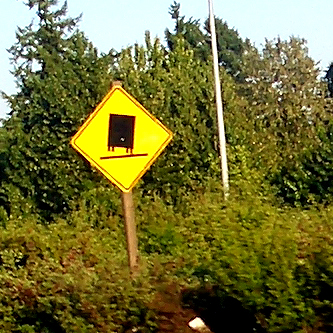This outdoor image captures the side of a road featuring a prominent caution sign positioned slightly left of center. The sign is mounted on a brown, 4x4-inch wooden post and displays a yellow, diamond-shaped symbol set on its diagonal axis. Its outer edge is bordered by two black stripes. The central graphic depicts a flat road with a box-like vehicle on four wheels tilting to the side, serving as a clear warning to drivers about the potential for uneven road surfaces that could cause trucks to tip over.

To the right of the caution sign stands a tall, silver pole, likely supporting a streetlight, with a round and circular structure. The foreground is dotted with low bushes, areas of red bark dust, and a small white spot that appears to be litter. Behind the silver pole, a mix of deciduous and evergreen trees forms a lush backdrop. The deciduous trees are fully leafed out, adding to the sense of depth and natural beauty in the scene.